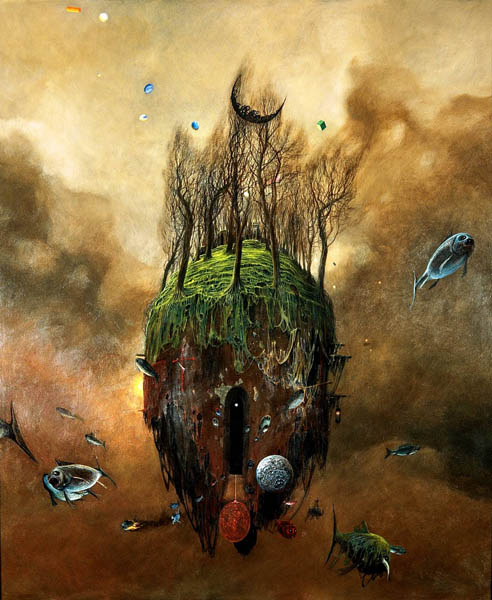The image is a surreal and abstract painting depicting a scene that seems to be either computer-generated or hand-drawn, set against a brownish-orange sky filled with smoky fires. The focal point is a floating island in the middle, which features a huge arched doorway leading into darkness. The island's base resembles a large stump with roots extending downwards, and its top is covered in lush green foliage and multiple trees. Among the treetops, there is a small crescent moon or possibly a tiny brown moon. Surrounding this island are various abstract elements, including strange, menacing little fish-like creatures, flying cubes, and spheres. Near the bottom of the image, there appear to be two globe-like objects that resemble planets. Vivid flashes of color and different floating objects add an extra layer of surrealism to the scene, while the barely visible sun and its rays peek out from behind the island.